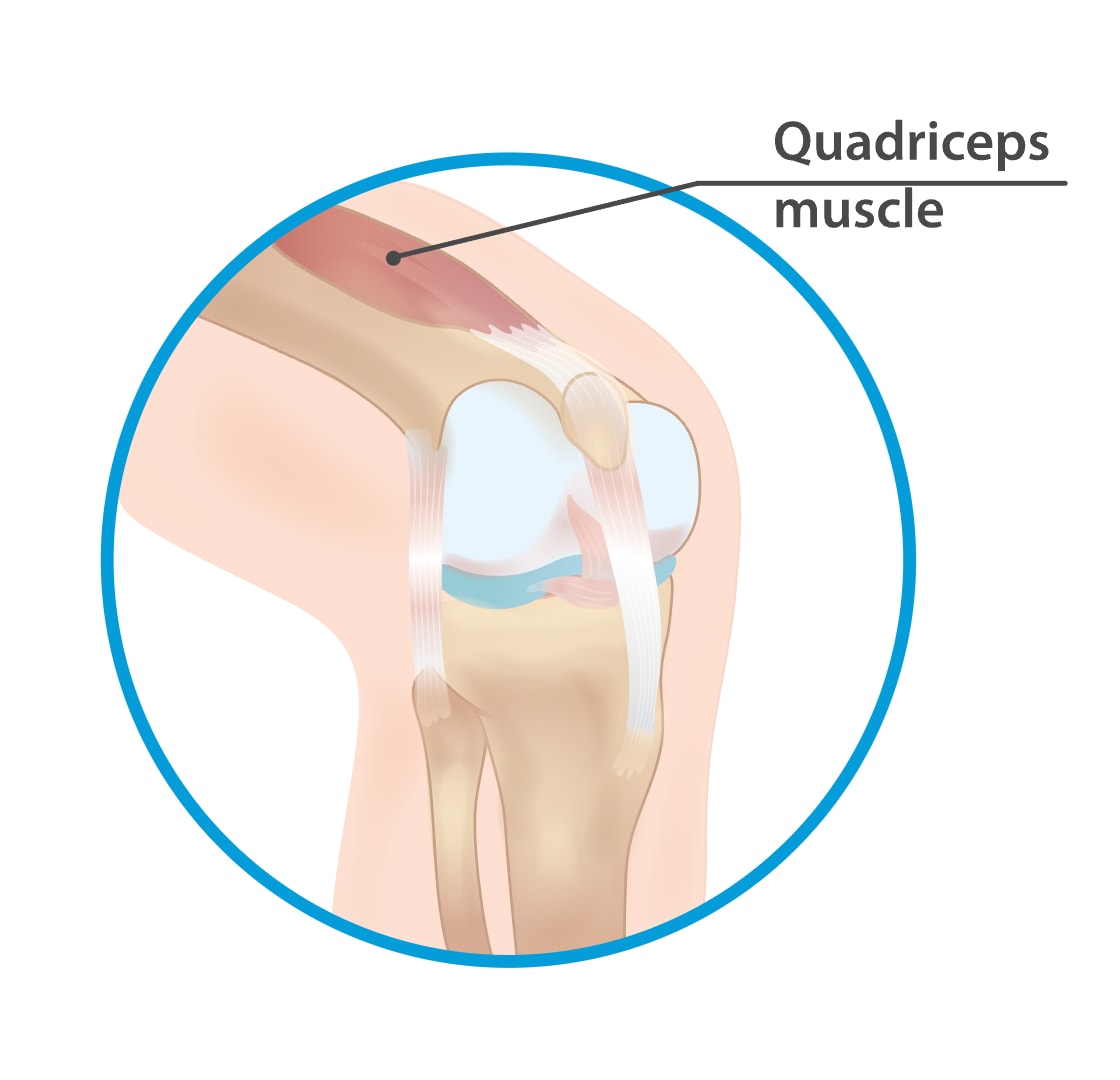The image is a detailed medical diagram of a human knee, featuring a bent knee in a zoomed-in cutaway view, encircled by a thin blue border. The white background highlights the illustration's soft color palette, achieved without significant shading or outlining. Prominently labeled "quadriceps muscle" in a light black font, the text is divided by a line, with "quadriceps" positioned above and "muscle" below. This line extends into the circular frame, pointing precisely to the quadriceps muscle in the thigh area, depicted in dark brown. Surrounding this main focus, the diagram intricately displays the layers of the knee, including pink-hued outer skin, cartilage, ligaments, and the knee bone in shades of brown and white. This comprehensive, animated representation serves as an educational tool for medical or physical fitness purposes.